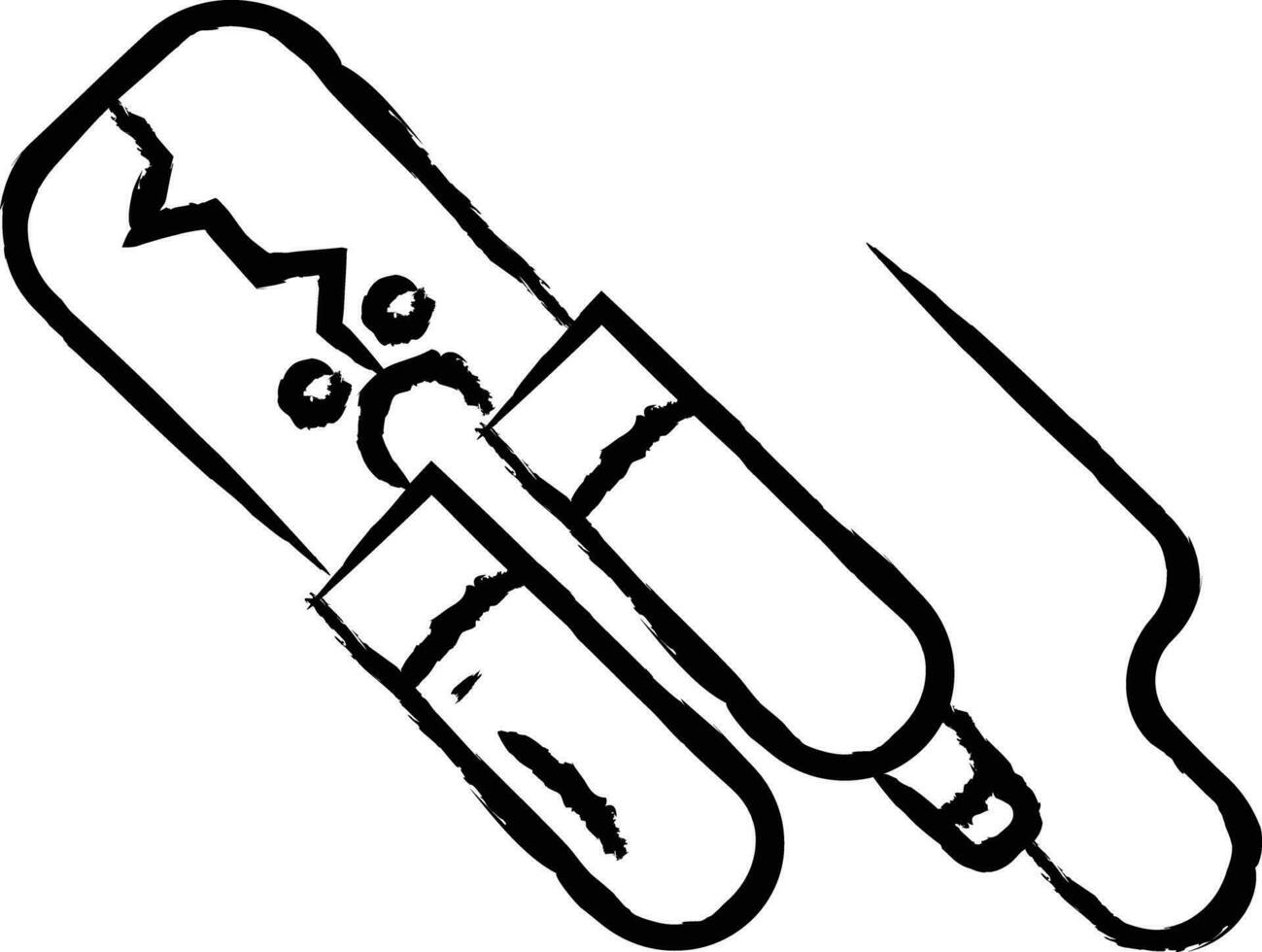The image features a black and white, digitally drawn graphic set against a stark white background, likely created with black brushstrokes. Central to the illustration is a tool-like object resembling a pair of shears or jumper cables, rotated 45 degrees counterclockwise. The top section is rectangular with rounded edges, containing two bolts that look somewhat like eyes. Below this section, two handles extend outward, with the left handle distinctly marked by a thick, black line adding a 3D effect. Notably, a wire emerges from the bottom right handle, looping around, which gives the tool an electronic rather than purely mechanical appearance.